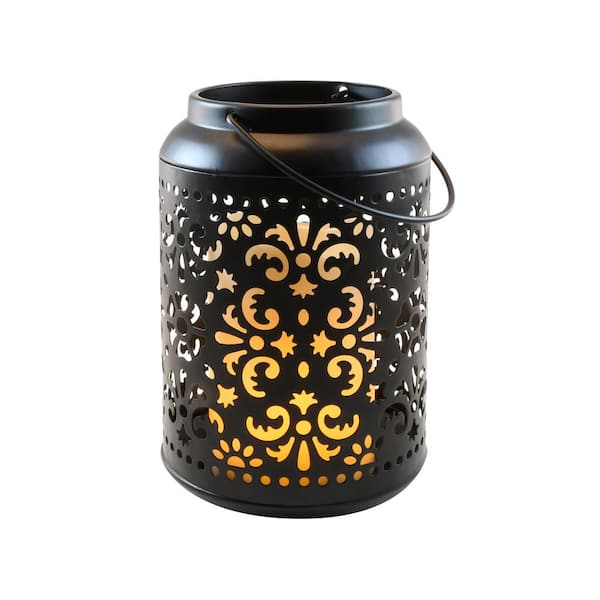In the center of the image, there is a black metallic candle holder with intricate perforation patterns that allow light to shine through. The cylindrical candle holder, with a solid bottom and top cap, features a decorative design with about 60% metal and 40% holes in various shapes and sizes. A curved metal handle drapes to the side, suggesting it can be carried but primarily serving a decorative purpose. Inside the container, a glowing yellow candle illuminates the abstract patterns, casting a warm, golden hue. The candle holder is set against a plain white background, emphasizing its intricate design and the soft glow emanating from within.